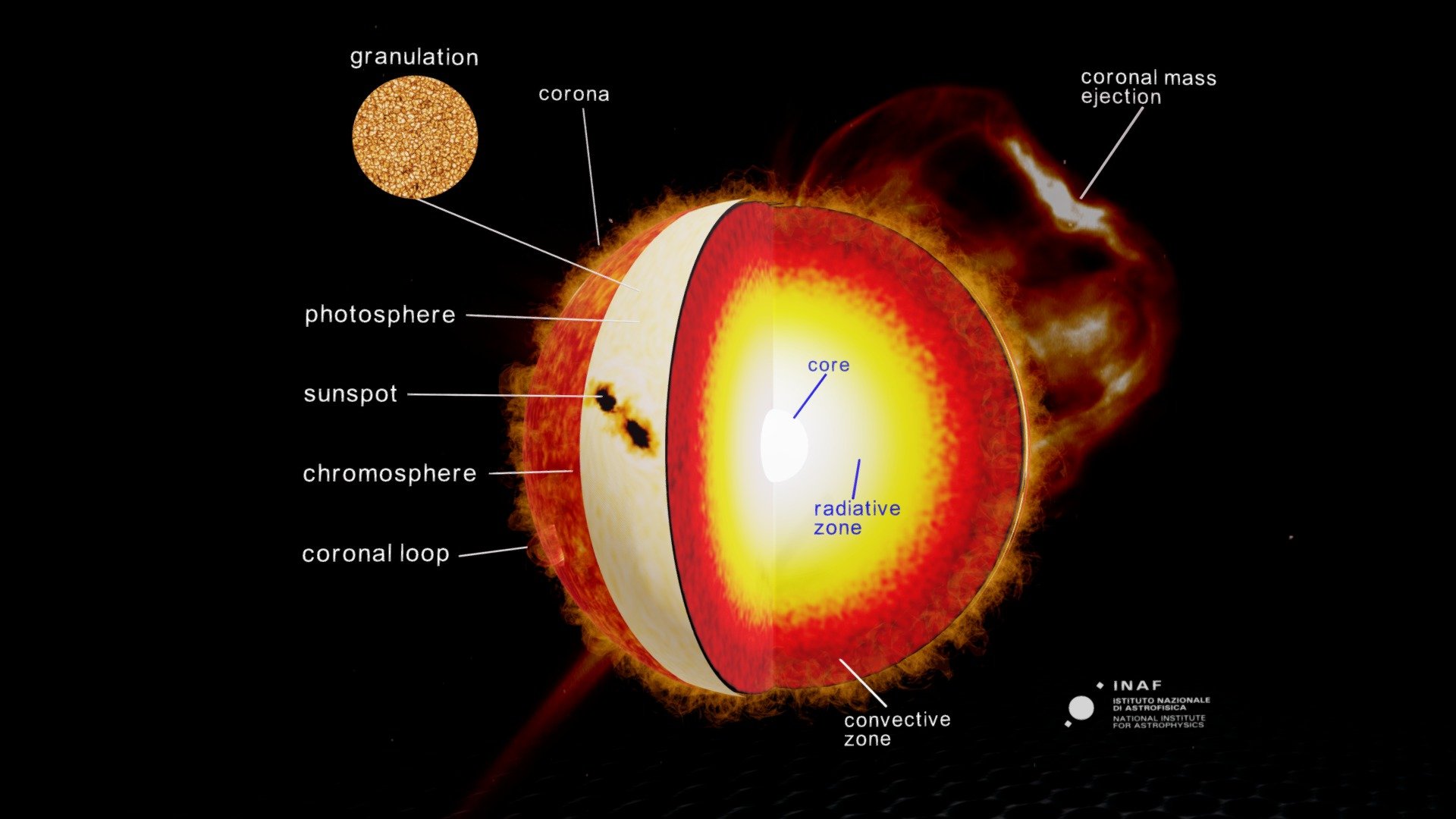The image is a detailed diagram of the Sun, set against a black background, illustrating its multi-layered structure through cutaways. At the center, a bright white core is labeled "core" in blue text with a white line pointing to it. Surrounding the core, the yellow area is labeled "radiative zone," followed by an orange outermost layer labeled "convective zone." Various other sections are labeled with white text and lines, including the corona, photosphere, chromosphere, sunspots, and coronal loop. The upper right-hand corner features an illustration of flames, marked as "coronal mass ejections," while the upper left-hand corner displays a disc labeled "granulation." The sunspots are depicted as dark brownish-black areas on the photosphere. In the lower right-hand corner, there is a white text label "INAF," indicating Instituto Nacional de Astrofisica, along with its logo.